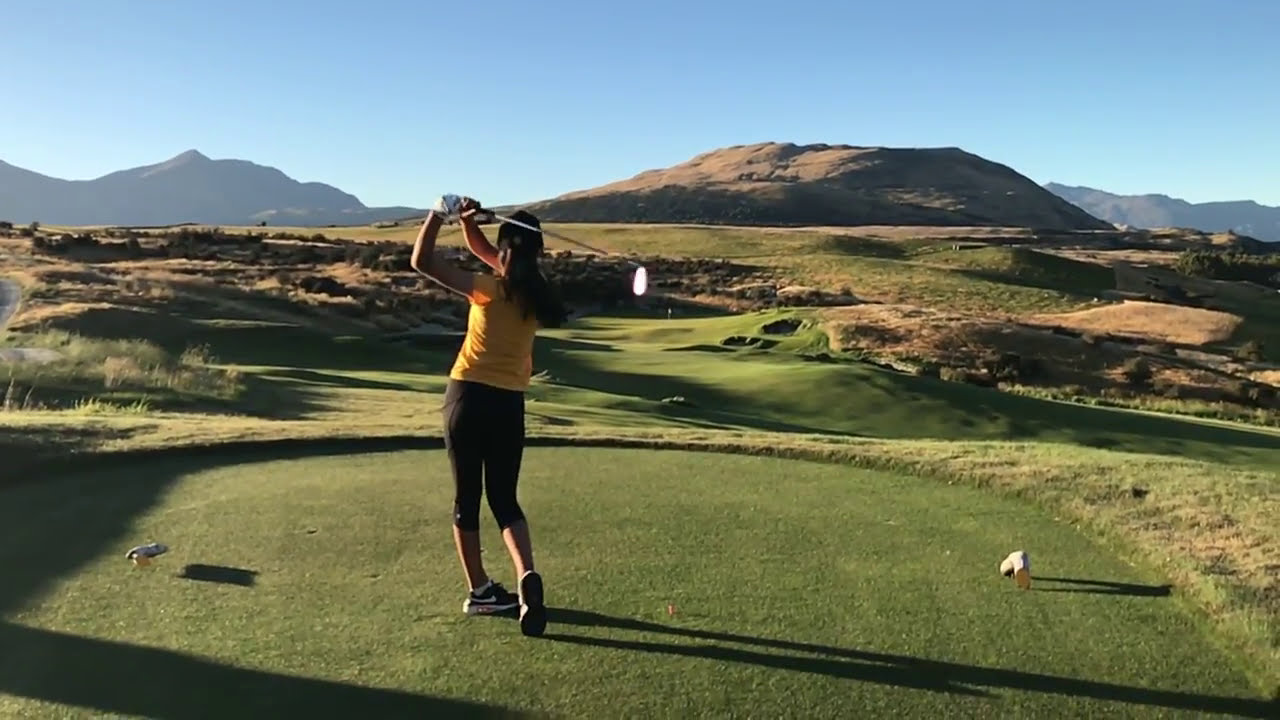In this vivid outdoor scene set on a flat, green tee box at the beginning of a lush, rolling fairway, a woman stands poised to tee off on a sunny golf course. The foreground features vibrant green grass and various golfing markers, with a paved path visible to the left. Wearing sneakers, black slacks, and a yellowish-orange shirt, the woman lifts her driver high behind her head in preparation for her swing. Her black hair cascades down past her shoulders. In the distance, tan and brown hills softly meld into a hazy, bright blue sky, adding depth and contrast to the image. The stillness of the distant flag and the surrounding tall grass underscore the calmness of the day, as the scene captures the essence of a serene midday golf experience.